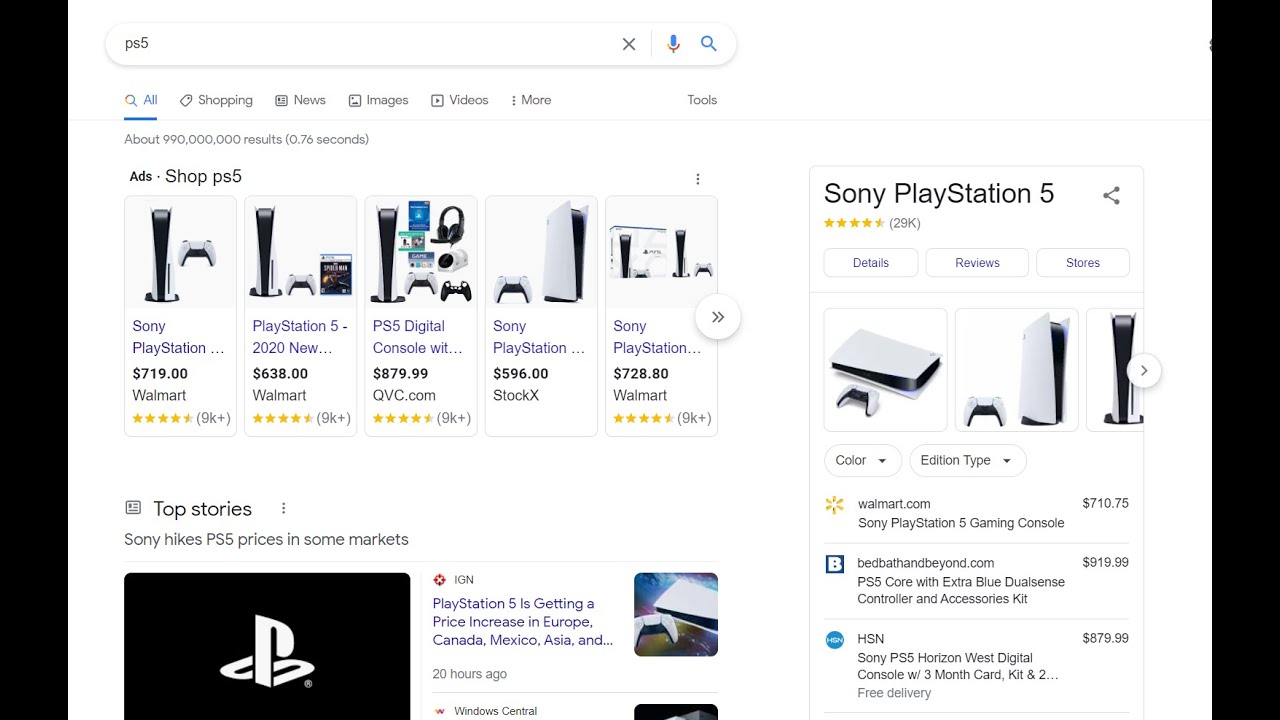The image is a horizontal, left-to-right screenshot from a smartphone, focusing on a search query for "PS5" on a web browser. The background is predominantly white, signifying a standard search engine interface with minimal distractions. The image is bordered vertically by thicker black edges, which frame the content.

At the top, the search bar is clearly visible, containing the query "PS5" along with the typical icons for voice search (microphone), clearing the search (X), and initiating the search (magnifying glass). Below the search bar, the active navigation is highlighted in blue, allowing the user to switch between different categories like "All," "Shopping," "News," "Images," "Videos," and "More." The "Tools" option is also available, suggesting further refinement of search parameters.

The search results show a breakdown of various content related to the PS5. Immediately below the search navigation, there are advertisements for purchasing the PS5, followed by "Top Stories" with the highlight being "Sony hikes PS5 prices in some markets," complete with an icon. Recent news articles are listed along with timestamps indicating their freshness.

On the right-hand side, a detailed information box provides an in-depth look at the Sony PlayStation 5. This box includes the average star rating, number of reviews, and product details. It features thumbnail images of the console and options to select the color or edition. Additionally, it lists retailers like walmart.com, with brief descriptions and pricing details for the PS5, making it easy for a potential buyer to find purchasing options.

Overall, the image captures the essence of an online search experience for the PS5, emphasizing both search results and detailed product information.